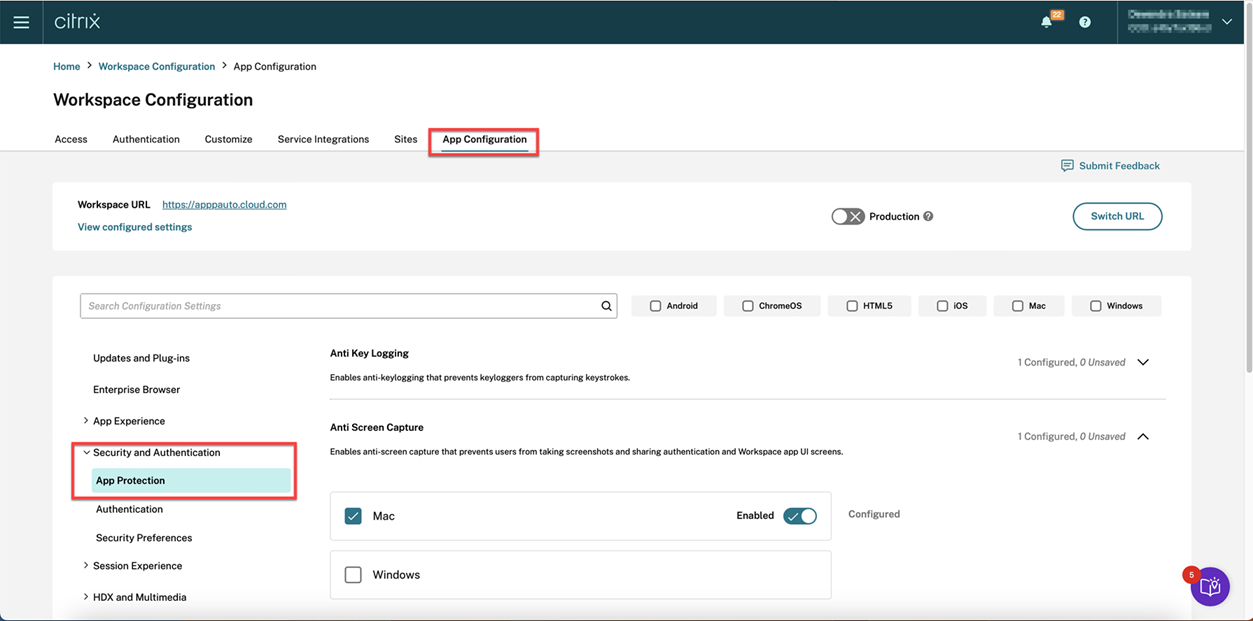The image appears to be a screenshot of a Citrix workspace configuration website. At the very top, a navy blue bar features the word "Citrix" in a whitish-blue font next to three horizontal lines, typically indicating a menu. Adjacent to this, there is a bell icon highlighted with an orange box, followed by a circular icon containing a question mark. 

Below the bar, a section with obscured or privacy-blurred information displays a mix of letters and numbers. Directly beneath it, a navigational menu includes options labeled "Home," "Workspace Configuration," and "App Configuration." 

The "Workspace Configuration" section unfolds into several submenus: Access, Authentication, Customize, Service Integrations, and Sites, highlighted by a surrounding red rectangle. The "App Configuration" section follows, with options to "Submit Feedback" and view the "Workspace URL," displaying a specific address. A button within an oval labeled "Production" sits next to the "View Configured Settings" option.

A search bar accompanied by a magnifying glass icon allows for configuration settings search. Below this, gray boxes categorize operating systems as "Android," "Chrome OS," "HTML5," "iOS," "Mac," and "Windows."

Further down, additional menus include "Updates and Plugins," "Enterprise Browser," "App Experience," "Security and Authentication," and "App Protection," with the "App Protection" section demarcated by a red box. Under it, subcategories like "Authentication," "Security Preferences," "Session Experience," "HDX," and "Multimedia" are listed. Specific focus is given to "Anti-Key Logging," which prevents keyloggers from capturing keystrokes, showing "One Configured, Zero Unsaved." The "Anti-Screen Capture" feature is similarly detailed, preventing screenshot taking and sharing within the workspace UI, also marked as "One Configured, Zero Unsaved."

A white box labeled "Mac enabled" is checked, and an unchecked "Windows" option lies below it. Finally, a purple-and-white circular icon with a red circle inside is present at the bottom of the screenshot.